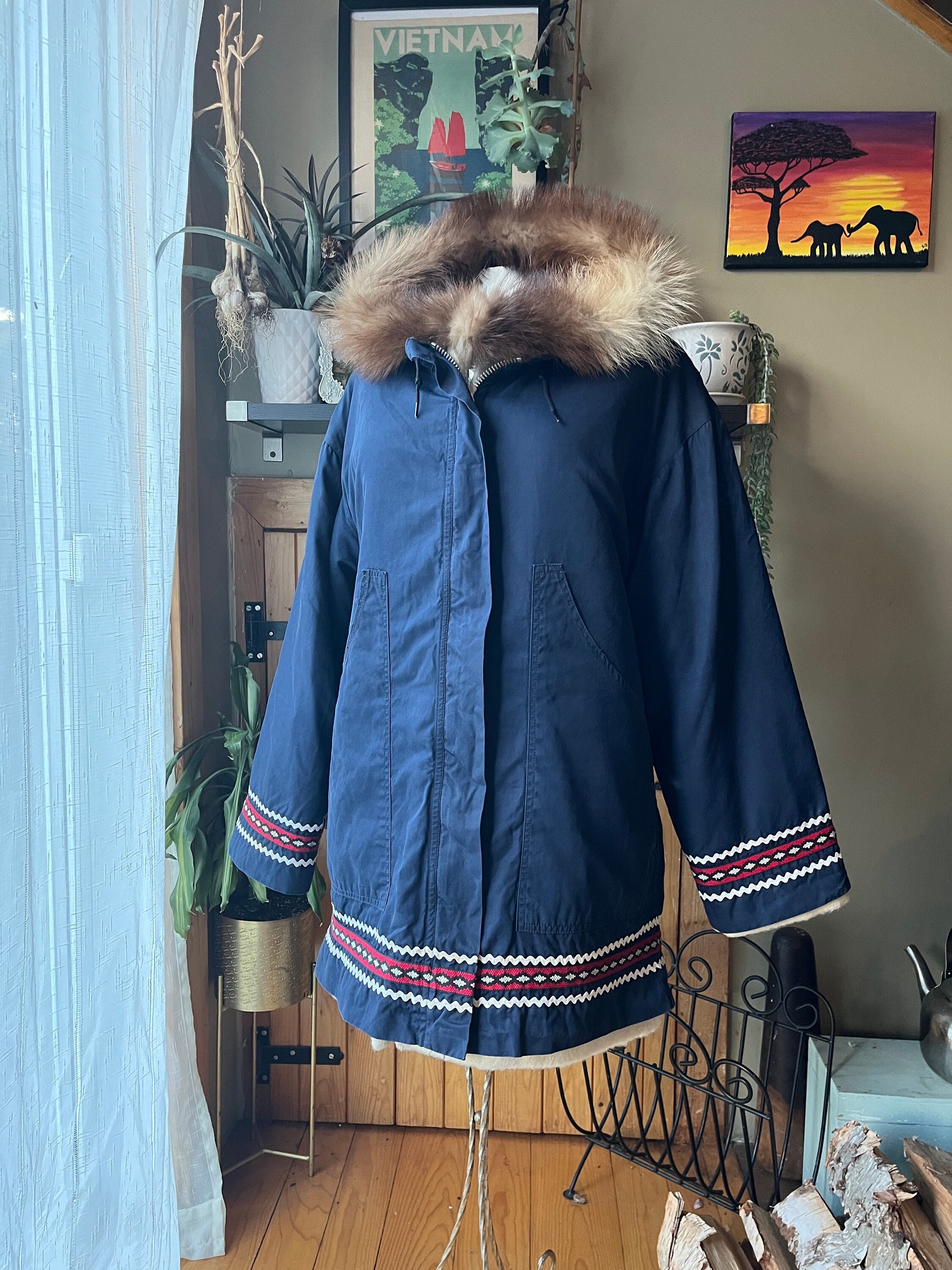In the center of this detailed room photograph, a dark blue jacket with a fur-lined hood is displayed on a dressmaker's dummy. The jacket showcases intricate detailing, including a jagged white zigzag pattern around the cuffs and hem. A pink ribbon runs through the middle of the garment, emphasizing its design. Behind the jacket, a small portion of the dummy's neck or head is visible through the hood.

The background reveals a green wall adorned with two pieces of art: a vibrant poster of Vietnam at the top center and a sunset painting featuring two elephants to the right. An array of elements fills the space, including a plant seen in the left corner of a shelf behind the jacket, and a glimpse of a short wooden door just behind it. A stack of firewood is placed in the lower right corner, adding a rustic touch. The floor is made of wooden planks with a nice brown color, and a white curtain allows natural light to filter into the room from the left side. This thoughtfully decorated space captures a mix of natural elements and global influences.